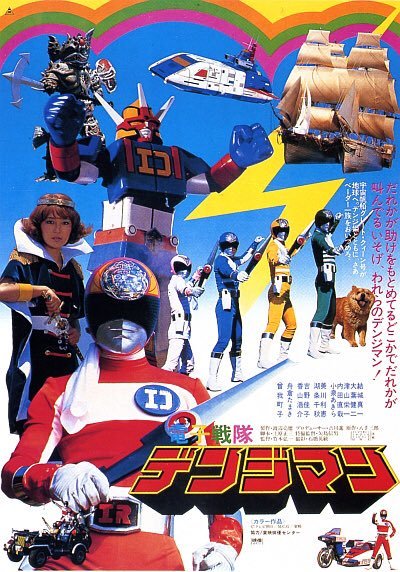The image is a vibrant and detailed poster of the popular Power Rangers movie set against a multicolored backdrop. Dominating the foreground is the Red Ranger in his red and white suit, brandishing a small sword with the letter "D" prominently displayed on his chest. Flanking him are the other Rangers: the Pink Ranger, the Blue Ranger, the Yellow Ranger, and the Green Ranger, each similarly armed with small swords. To the left of the Rangers, a woman in a uniform with a simple crown-like band around her head is poised to draw her sword. Behind them, the colossal Megazord looms, adding to the dramatic effect.

In the background, on the left, a monstrous figure with a spear adds a touch of menace, while to the right, a red, blue, and white flying craft hovers mid-air. On the top right corner, two old-fashioned ships with sails appear to be ready for adventure. Completing the scene, there is a chow dog standing next to the Blue Ranger, and at the bottom right, a red ninja poses beside a red, white, and blue motorcycle. The entire image, punctuated with red text at the bottom, exudes action and excitement, characteristic of the Power Rangers franchise.